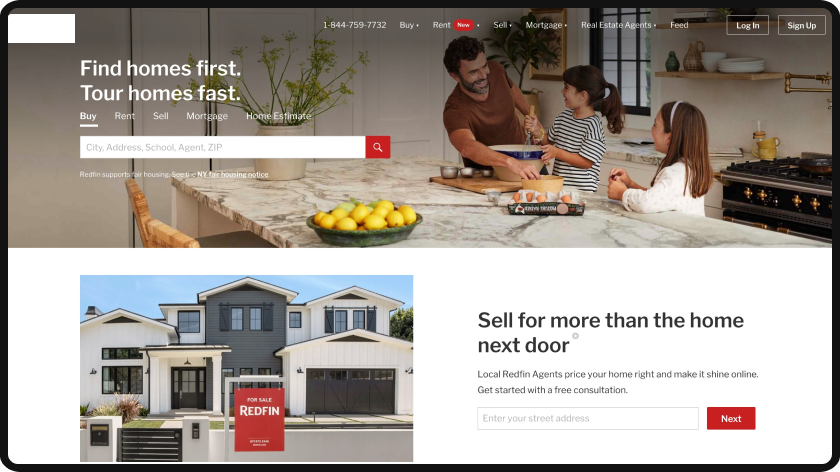On the presented webpage, a heartwarming family moment unfolds within a vibrant kitchen scene. At the center stands a father, smiling warmly at his child, as he reaches towards a wooden bowl. Wearing a brown t-shirt that reveals his hairy arms and clean-shaven face, he radiates joy and engagement. His short brown hair adds to his neat appearance. 

Adjacent to him, his daughter, with her shoulder-length black hair tied up in a ponytail, mirrors his joy. With a light complexion and a bright smile, she stirs contents in a large tan mixing bowl accented with a dark blue band, placed atop a wooden cutting board surrounded by several silver bowls. Eggs are positioned to her right, emphasizing the family’s culinary activity.

Next to her, another daughter joins in the blissful interaction, both of her hands placed on the white marble countertop which features intricate bands of dark gray, light gray, and tan hues. Her brown, shoulder-length hair is adorned with a headband, and she too wears a gleeful expression, clad in a long-sleeved white top. Their shared laughter highlights the strong familial bond.

Behind the family, the kitchen walls are painted a crisp white, providing a clean backdrop. A stove and a door with a window are visible to the right, balancing the homely yet detailed environment.

The webpage design features multiple user interface elements. Below the family scene:

- There are illustrations of various buildings, one stacked with a 'For Sale' sign by Redfin.
- A bold black headline encourages users to "Sell for more than the home next door", accompanied by a succinct description of Redfin's consultation services.
- An input box prompts visitors to enter their street address, followed by a prominent red 'Next' button.

At the top of the page, a navigation bar includes clickable options for "Buy", "Rent", "Sell", "Mortgage", and "Real Estate Agents". Additional elements include a prominent 1-844-759-7732 contact number, and buttons labeled 'New', 'Login', and 'Sign Up'. 

Further left of the family are decorative elements including a bowl of lemons in a green border, and a planter featuring dark and yellow-green leaves blends seamlessly within the scene. Above this is the bold text, "Find Homes First" and "Tour Homes Fast," emphasizing the quick search and tour capabilities of the site, supported by clickable categories such as "Buy”, “Rent”, “Sell”, "Mortgage", and "Home Estate".

The search bar, styled as a white and gray rectangle, offers filtering options by City, Address, School, Agent, and Zip, ending with a red square icon of a magnifying glass. Below this, Redfin's commitment to fair housing is highlighted with a note on the NY Fair Housing Notice, showcasing their adherence to housing rights.

This comprehensive scene intricately combines family warmth with detailed navigational elements, embodying both personal connection and practical usability on the Redfin platform.